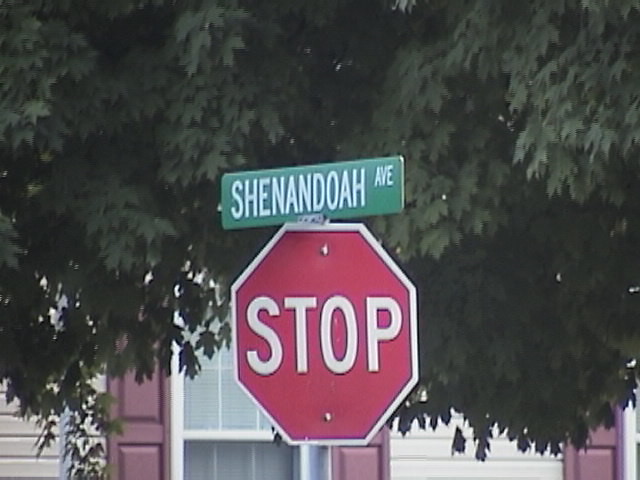An outdoor scene captured in soft gray light showcases a classic red octagonal stop sign prominently centered in the frame, bearing the word "STOP" in bold white letters. Above the stop sign, a green rectangular street sign reads "Shenandoah Ave." To the right, the front wall of a house is partially visible, featuring off-white siding, burgundy shutters, and two partially visible windows. The background is dominated by the dense, leafy canopy of a mature maple tree, its lush green leaves providing a natural backdrop that contrasts with the man-made elements of the scene.